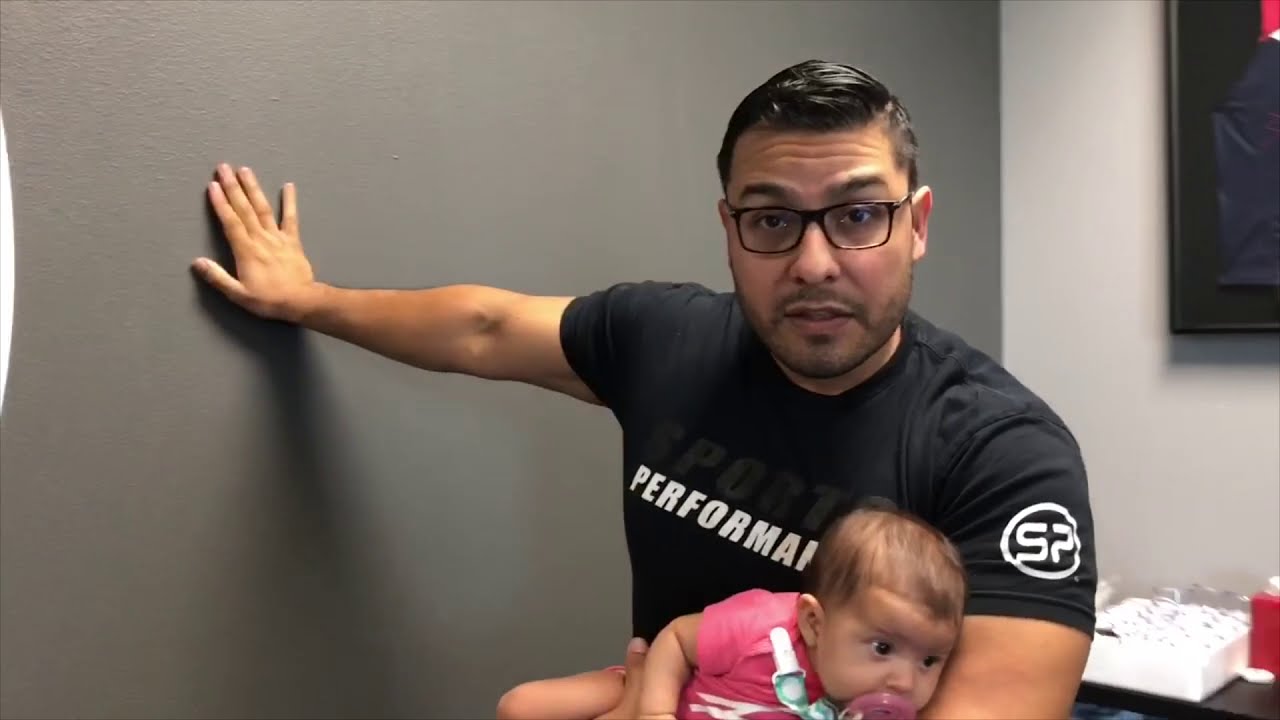The photograph captures a striking moment between a father and his infant daughter. The father, positioned slightly off-center to the right, is wearing dark square-rimmed glasses and a sleek, black "Sports Performance" shirt, which features a small logo with the initials "SP" on his left sleeve. His shiny, gelled black hair adds to his well-groomed appearance. He stares intently at the camera while bracing his right hand against a gray wall. 

In his left arm, he cradles his daughter, who is dressed in a pink outfit with a pink pacifier clipped to her shirt. The baby, with a small amount of hair, is nestled comfortably in the crook of his elbow, looking slightly downward.

The background reveals a mix of domestic elements. To the right of the father, the wall transitions to white, with a partially visible picture frame intruding into the upper right corner. Below this, a white changing table or surface is seen, adorned with a red tissue box and a white tray holding some clear bottles, possibly baby wipes. This careful blend of details paints a vivid picture of a tender, yet everyday, moment in a family's life.